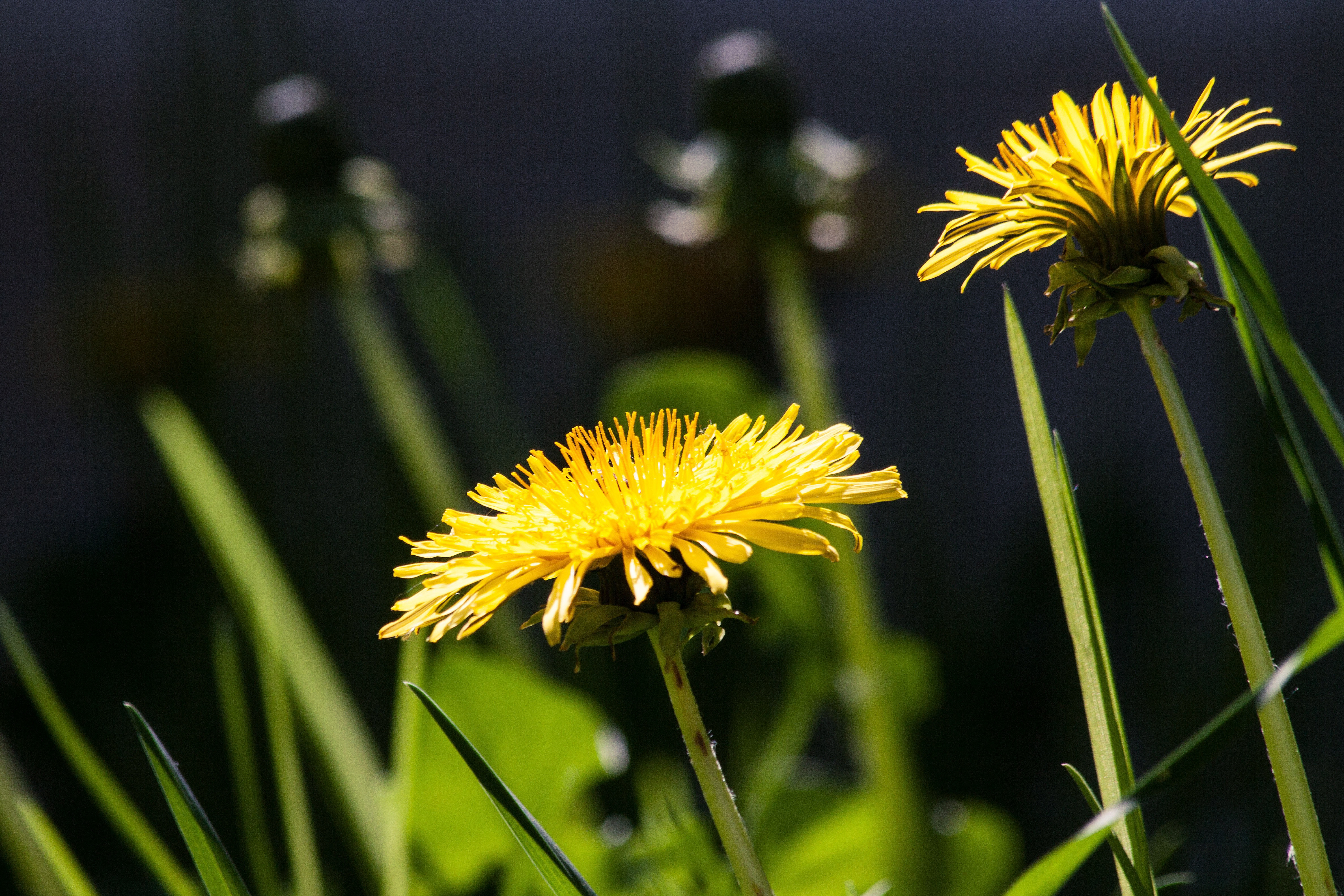The image depicts a detailed, close-up view of two fully-bloomed yellow dandelions set against a blurred, dark background that hints at more flowers and vegetation. The flowers are the focal point, with their thin, rounded yellow petals standing upright in the middle and laying flat on the sides. Each flower is supported by a green stem, which appears greener and more vivid towards the front of the image. Small green leaves emerge from the sides, and delicate droplets of water can be seen clinging to the stems. The background has a moody, dark blue hue, suggesting it might be evening or heavily overcast, emphasizing the brightness and clarity of the flowers in the natural daylight setting. Despite the close focus, there is a noticeable presence of more grass and possibly flowers in the backdrop, which is artfully blurred to enhance the sharpness and beauty of the two prominent dandelions in the foreground.